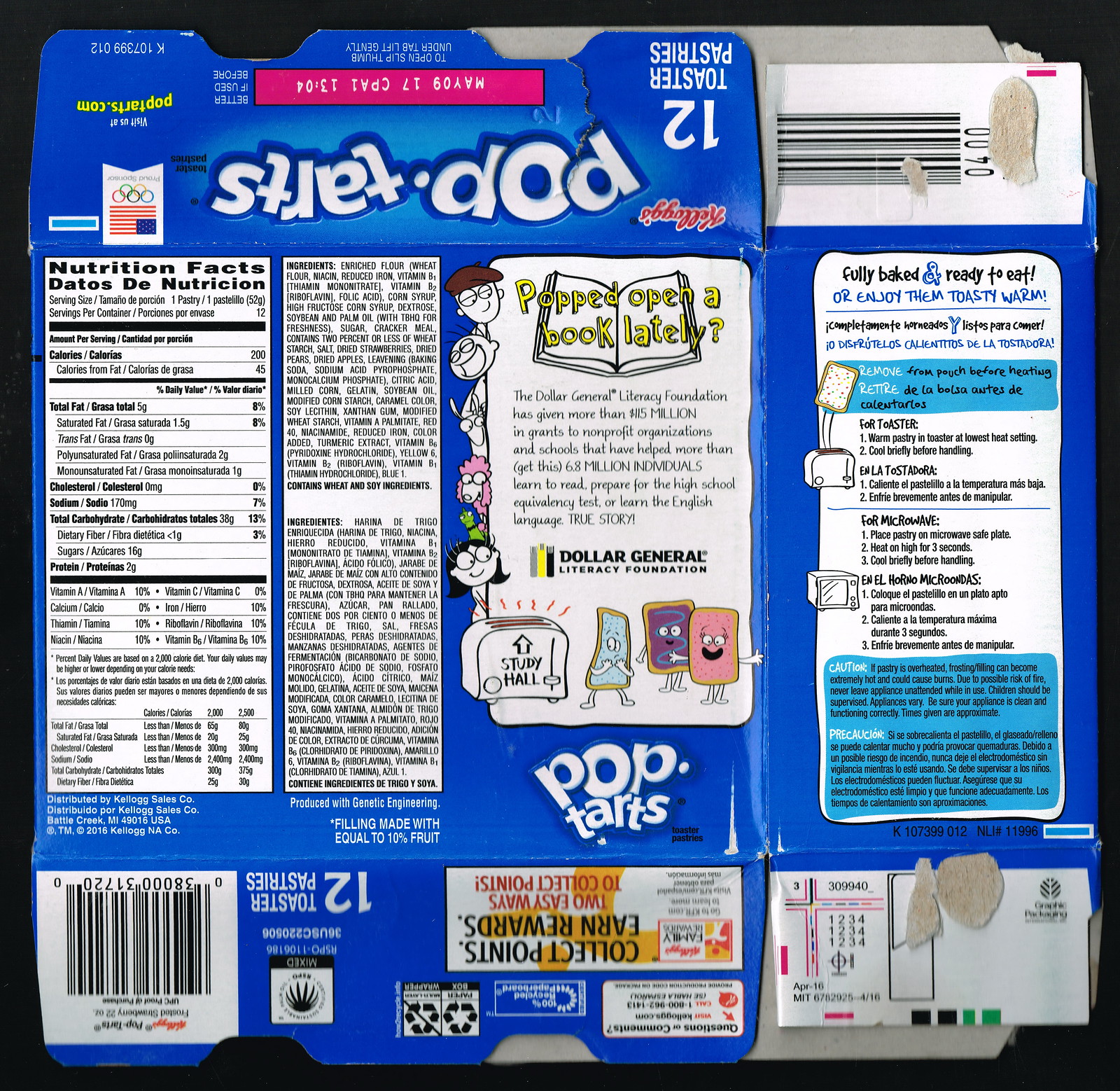This detailed caption incorporates key elements from all three descriptions:

In this image, we see the back view of a completely flattened, empty Pop-Tarts box, previously containing 12 toaster pastries. The box is primarily blue, and despite being laid flat, key elements are still visible. At the top of the image, "Kellogg's Pop-Tarts" is written, with the Kellogg's logo in red. The expiration date is May 9th, 2017. There’s also an American flag symbol accompanied by circular logos and a white square. Nutritional information is provided in both English and Spanish. To the left, we see a barcode and various recycling logos. There's a section with instructions on how to prepare the Pop-Tarts in a toaster or microwave. Notably, a large banner at the bottom of the box, displayed upside down due to its flattened state, says "Collect Points, Earn Rewards" and mentions two easy ways to collect points. Additionally, there is a promotional message about partnering with Dollar General to encourage children to read, featuring the slogan "Popped Open A Book Lately?"